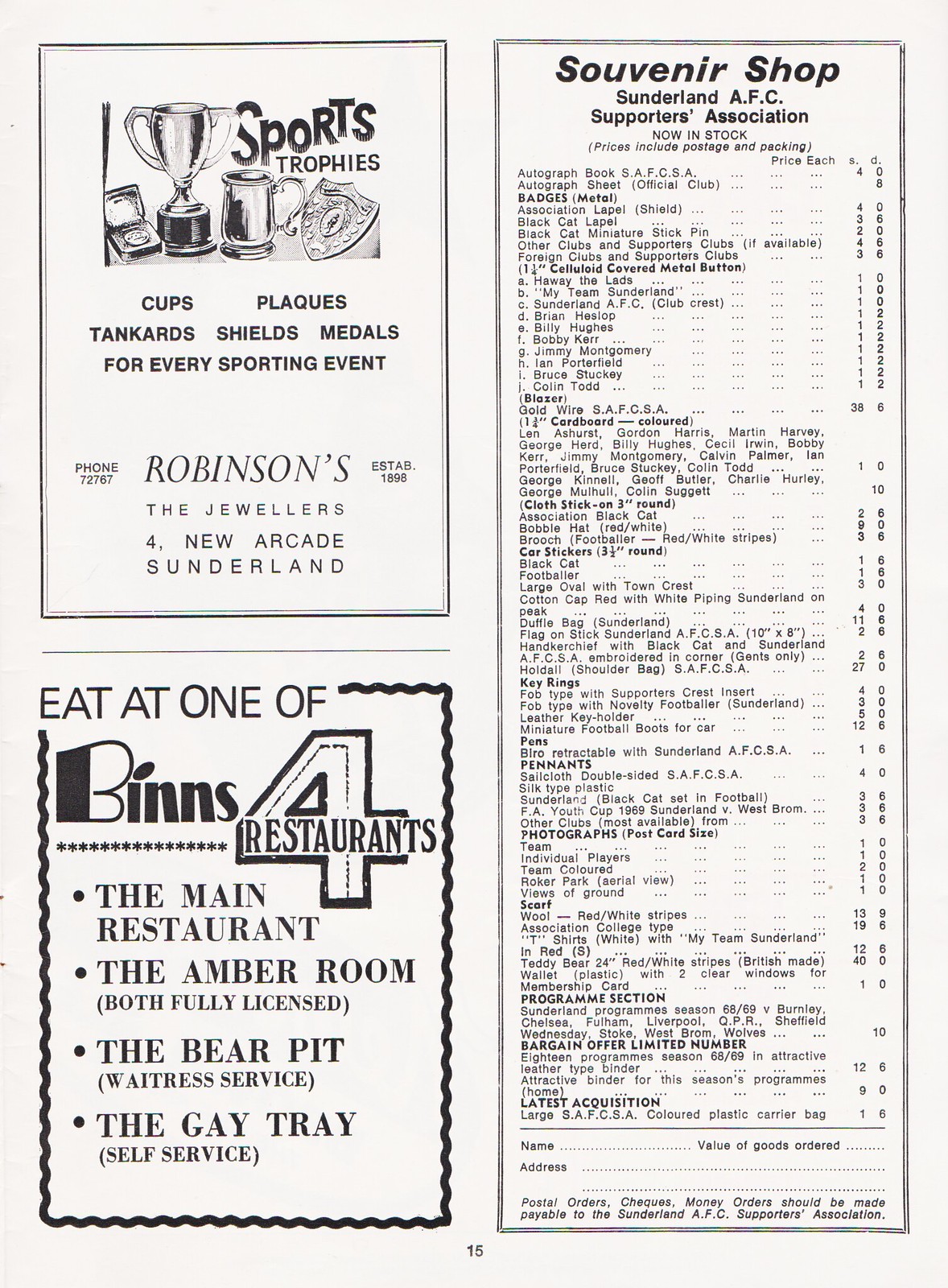The image depicts a black-and-white vintage program page, labeled as page 15 at the bottom, in portrait orientation. The background of the page is white and it is divided into three sections, with two on the left and one large section on the right.

On the top left section is an advertisement for Robinson's, the jewelers from Sunderland, established in 1898. The ad features the heading "Sports Trophies" accompanied by various trophy icons. Below the icons, it lists different types of trophies available: cups, plaques, tankards, shields, and medals suitable for every sporting event. The contact detail, "Phone 72767," is also included.

Directly beneath this ad is another advertisement for Ben's Four Restaurants. A prominent number "4" with the word "restaurants" inside it draws attention. The ad invites readers to "Eat at one of Ben's Four Restaurants," detailing the different dining options: The Main Restaurant (The Amber Room, fully licensed), The Bear Pit (waitress service), and The Gay Tray (self-service).

On the right side of the page is a section titled "Souvenir Shop - Sunderland AFC Supporters Association." This section lists various memorabilia available for purchase, such as autograph books featuring names like Jimmy Montgomery, Bruce Stuckley, and Colin Todd, with prices ranging from $1 to $4. There is also mention of badges, pennants, and photographs, presented in a detailed manner with prices. This section includes an order form at the bottom, allowing customers to fill in their name, value of goods ordered, and their address, with the note that prices include postage and packaging.

Overall, the page combines illustrative advertising for sporting trophies and dining options with a detailed product listing for Sunderland AFC supporters' souvenirs, maintaining a cohesive vintage publication style throughout.